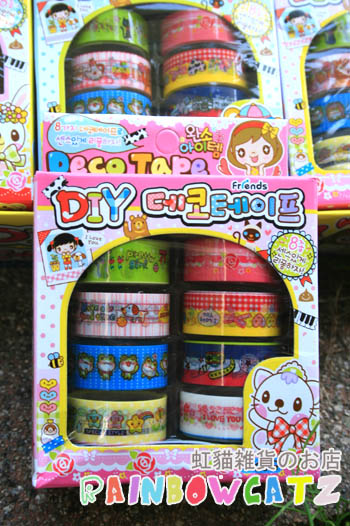This vibrant photograph showcases a brightly colored box of washi tape labeled "DIY," followed by Korean text, with "FRIENDS" written prominently at the top. In the bottom right corner, the words "RAINBOW CATS" appear in rainbow colors, accompanied by Japanese text above in brown. The packaging features eight distinct rolls of washi tape, each with a unique design: one green, one with orange and pink stripes, a blue roll adorned with frogs, a yellow roll with multicolored stars, pink, red, white, and blue tape, another yellow and red roll with red polka dots, and a final roll that says "I LOVE YOU" with hearts on a white-bordered background.

Above this main featured box, there are three additional boxes of the same washi tape set, all arranged neatly on a marble-effect surface, reinforcing the childlike and playful nature of the product geared towards crafts. The packaging is colorful—red, blue, yellow, and pink—and includes a distinct tab that says "DECO TAPE" with an illustration of a brown-haired girl wearing a red hat and sporting a yellow butterfly near her head. The background depicts a row of these DIY Rainbow Cats kits, indicating a bright and cheerful theme, making it evident that the design is whimsical and suitable for children.